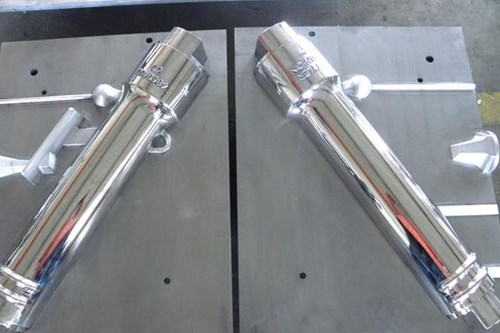The image depicts a sterile, scientific laboratory setting featuring two metallic tube-like structures laid horizontally in the center of the frame. These tubes, likely constructed from steel, are mounted on large, rectangular metal plates that rest on a either concrete or marble surface. Each tube has a series of ringlets along its length, possibly for threading or securing purposes, and displays some unreadable text near the top, possibly indicating measurements or manufacturer details. The metal plates, symmetrical in design, have a series of eight symmetrically drilled holes with two at the top, two on the bottom, and one on each side, all arranged in a precise pattern. Additionally, on the right side of the image, there is a metal cone-shaped component tilted upwards to the left. The entire setup, viewed from either a straight-on or top-down perspective, suggests it could be some type of tool, instrument, or part of a larger apparatus, hinting at its utility in a laboratory or scientific application.